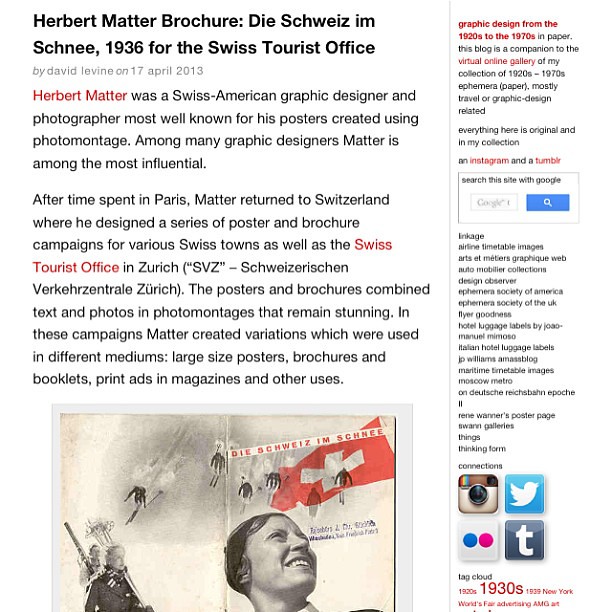The screenshot depicts a 2013 article by David Levine titled "Herbert Matter Brochure, Die Schweiz im Schnee 1936 for the Swiss Tourist Office." The article, posted on April 17th, delves into the impactful work of Swiss-American graphic designer and photographer Herbert Matter, renowned for his photomontage posters. A black and white image dominates the bottom of the screen, featuring vintage elements such as skiers on a mountain, a woman's face, and a soldier, all unified by a vivid Swiss flag in the top right corner. The layout suggests a website format with a white background and various sections, including tags and a search box. The article praises Matter's influential designs, created for the Swiss Tourist Office, describing them as stunning combinations of text and photos utilized in various mediums like posters, brochures, and advertisements.